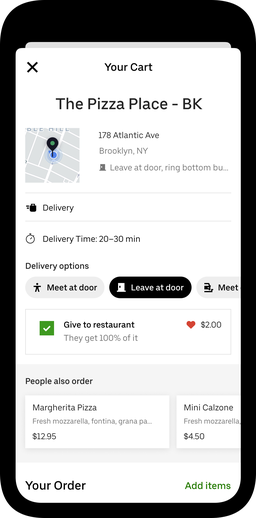The image is a digital screenshot of a smartphone, showcasing an online shopping cart interface from a pizza restaurant named "BK," prominently identified in bold text at the top. At the apex of the popup screen, there is an "X" icon in the upper left corner for closing the shopping cart interface. The header also displays the text "Your Cart."

Below the header, there is a small thumbnail image of a gray and white map with a pin indicating a specific location. Adjacent to this thumbnail on the right is the address: 178 Atlantic Avenue, Brooklyn, New York. Under the address, delivery instructions are partially visible, stating "Leave at door, ring, bottom, ba...".

Further down, there are identifiers related to the delivery, which include "Delivery," "Delivery time: 20 to 30 minutes," and delivery options: "Meet at door," "Leave at door," and a partially visible option "Meet...". The option "Leave at door" is highlighted in black, indicating it has been selected.

Directly below the delivery options, there is a section about tipping, featuring a green check mark next to the text "Give to restaurant." Beside this, there is a red heart icon accompanied by "$2.00."

Lower on the screen, there is a segment titled "People Also Order" followed by an ordering section at the bottom, displaying text "Your Order" and "Add Items."

Overall, the interface is designed for convenience, allowing users to manage their delivery preferences and tip options seamlessly.